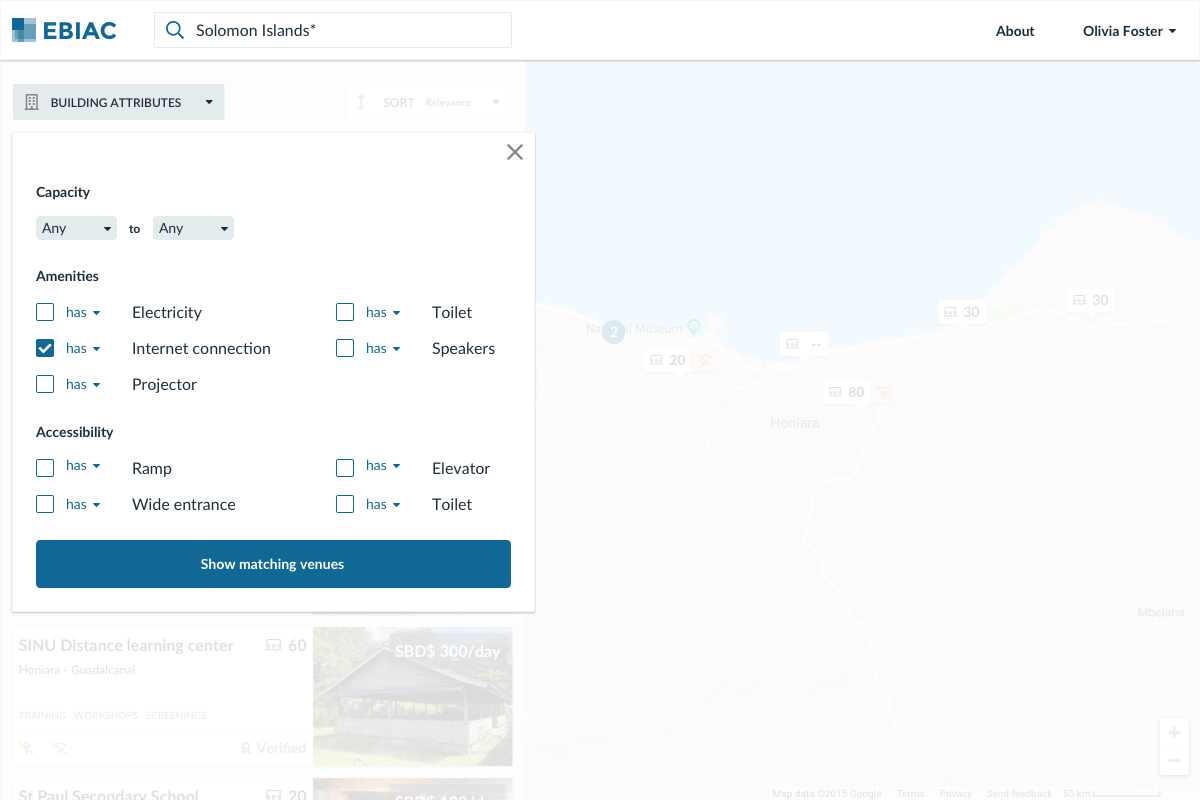The image depicts a website interface with a map subtly faded into the background, lending a contextual backdrop to the content. At the top of the page, a prominent white bar features the logo "EBIAC" in blue. Adjacent to the logo is a search bar with the text "Solomon Islands" entered, and an asterisk beside the 'S.' To the right, the words "About" and "Olivia Foster" are displayed in black, with a downward-facing arrow suggesting more options upon clicking.

A pop-up box is also present, offering extensive filtering options. In the top right corner of this box is an 'X' for closing it. The first section of the pop-up is labeled "Capacity" in bold, capital letters. It includes two dropdown boxes labeled "Any to" and "Any," enabling users to specify capacity preferences.

Below this, the "Amenities" section is prominently displayed in bold. Multiple check boxes are available for users to select specific amenities. Options listed include: "Has electricity," "Has Internet connection" (which is checked), "Has projector," "Has toilet," and "Has speakers." Notably, the word "Has" is highlighted in blue for each option, while the remaining text is in black.

The next section, labeled "Accessibility" in bold, offers similar checkboxes for features geared towards accessibility. These include: "Has ramp," "Has wide entrance," "Has elevator," and "Has toilet." As before, "Has" is in blue while the rest of the text remains black.

At the bottom of the pop-up box, there is a long white rectangle button which says "Show Matching Venues," suggesting it will display results based on the selected filters.